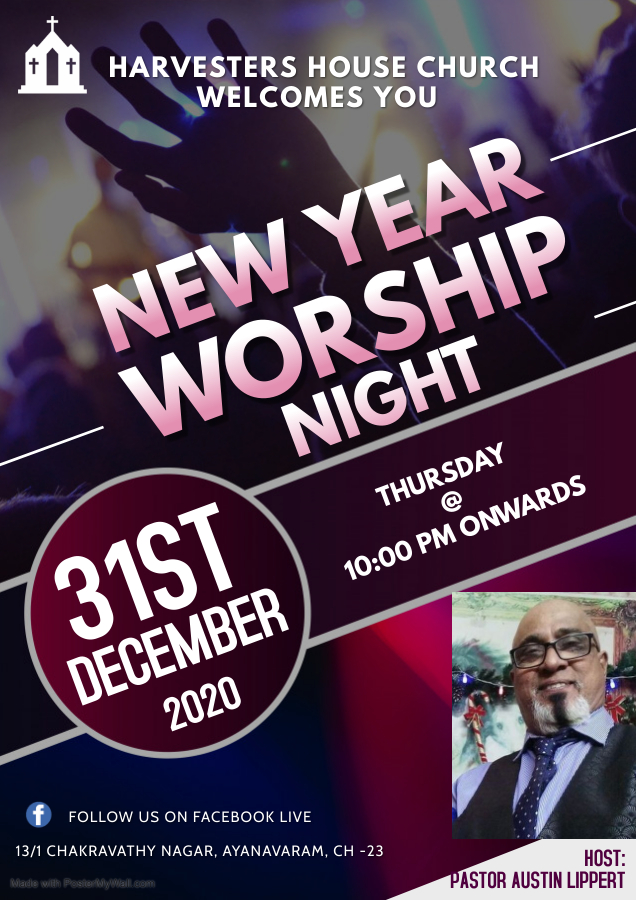The promotional poster for the Harvester's House Church welcomes you at the top with a white church icon featuring crosses and the text in bold letters. Below that, in bold diagonal pink and white text, it reads "New Year Worship Night." Adjacent to this, there is a circular emblem containing the date "31st December 2020" in white letters, along with a banner to the right that states "Thursday at 10 PM onwards." At the bottom right, there's a portrait of a man with brown skin, wearing glasses, a grey and black goatee, a shirt, vest, and a tie, identified as "Host Pastor Austin Lippert." To the bottom left, a Facebook icon with a white "F" inside a circle accompanies the text "Follow us on Facebook Live." The address is provided: "13/1, Chak Rafi Nagar, Ayo Faram, CH-23." The background of the poster features a blurred dark room with raised hands and a crowd, suggesting a lively worship environment. There's also an individual on stage playing the guitar, contributing to the worship atmosphere.